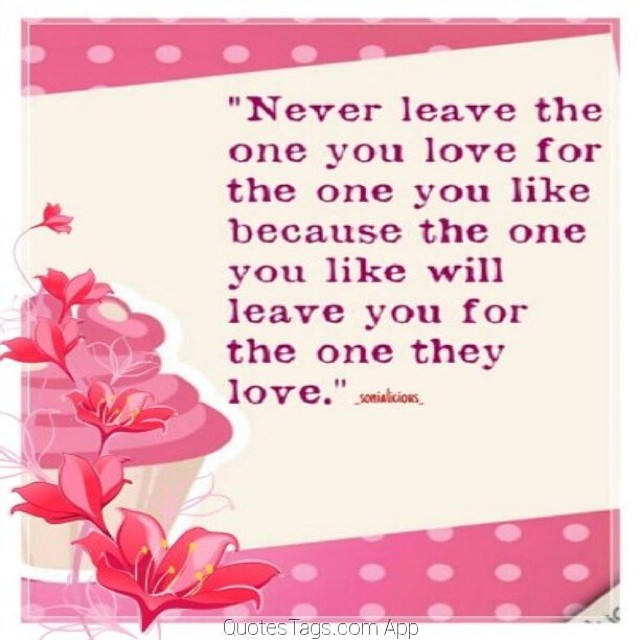The image is a motivational graphic featuring an inspirational quote framed within an asymmetric rectangle. The central quote says, "Never leave the one you love for the one you like because the one you like will leave you for the one they love," written in purple text. This quote is set against a predominantly white background that is tilted from lower left to higher right, giving it a dynamic orientation. 

This central white area is bordered by pink sections adorned with lighter pink polka dots at the top and bottom, adding texture and contrast. In the bottom left corner, there is a detailed graphic of a cupcake decorated with red flowers, adding a touch of whimsy to the overall design. The entire graphic is enhanced by a URL watermark at the bottom, attributing the quote to "quotestags.com app." The cohesive color scheme of pink, white, and red ties all the elements together into a visually appealing composition aimed at delivering a powerful message.